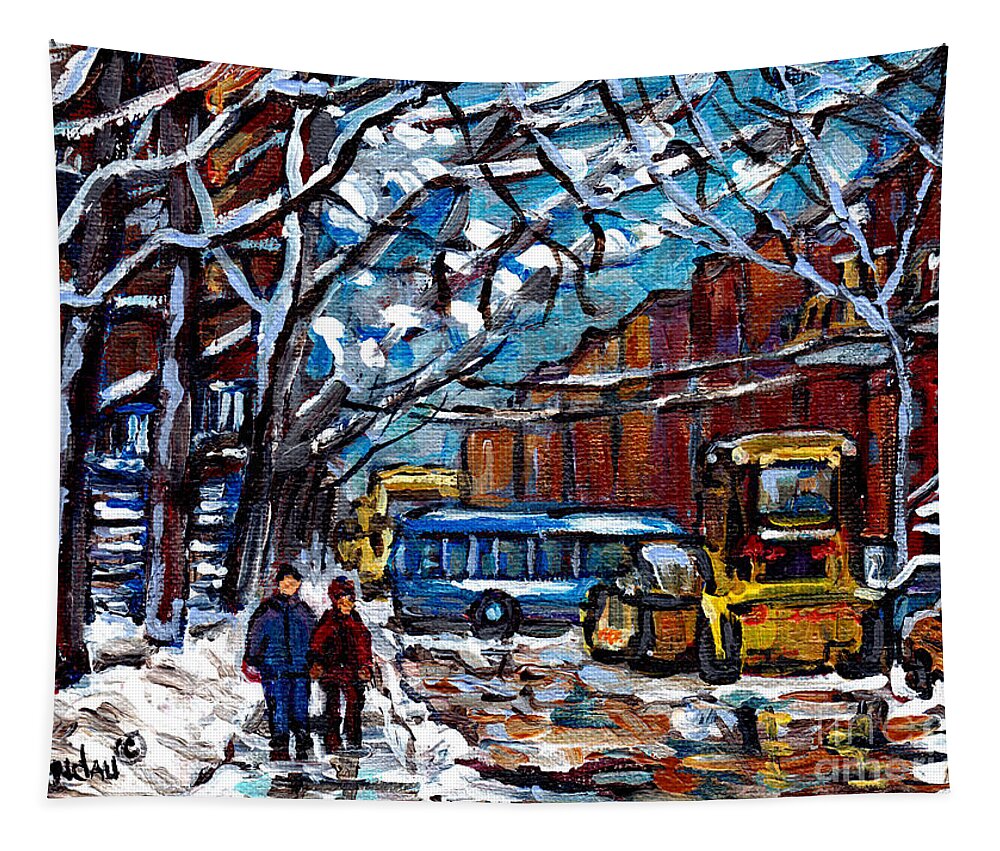This image features a primitive, impressionistic painting of a snowy winter city street scene. Dominated by simple outlines in black, the painting showcases a couple walking along a snowy pathway framed by large, leafless trees with snow-laden branches, against a backdrop of a clear blue sky. The couple consists of a taller figure in a blue tracksuit and a shorter figure in a red coat and black pants, devoid of detailed facial features. In the background to the right, the cityscape includes brownstone buildings, a rust-colored wall, and various vehicles: a blue bus, a plow, a yellow tractor truck, and a blue car. Snow blankets the entire scene, enveloping the buildings, ground, and trees. The artist's signature is faintly visible in the bottom left corner, though it’s difficult to discern, while a faint "Fine Art America" watermark appears in the bottom right.